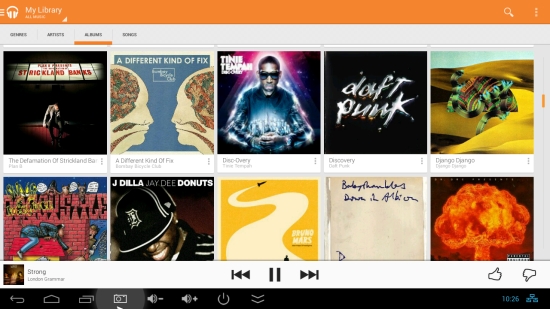This screenshot captures an interface from an unknown music application. An orange banner stretches across the top, featuring a white headphone icon next to the label "My Library." To the right of the banner, a white magnifying glass icon indicates the search function. The rest of the interface has a clean white background.

Below the banner, four navigation tabs are displayed: "Genres," "Artists," "Albums," and "Songs." The "Albums" tab is currently selected. 

The main section showcases a lineup of album covers and titles:
1. "The Defamation of Strickland Banks"
2. "A Different Kind of Fix"
3. "Disc-Overy"
4. "Discovery" by Daft Punk
5. "Django Django" by Django Django
6. "Strong" by London Grammar
7. "J Dilla" 
8. "JD Donuts"
9. "Bruno Mars"
10. "Baby Shambles"
11. An album with an illegible title featuring a striking image of a bright orange nuclear mushroom cloud and a parental advisory sticker at the bottom right corner.

At the bottom of the screenshot, the currently playing song is "Strong" by London Grammar. To control playback, there are navigational icons including a back button, a pause button, and a forward button. Additionally, thumbs up and thumbs down icons are available for user feedback on the song.